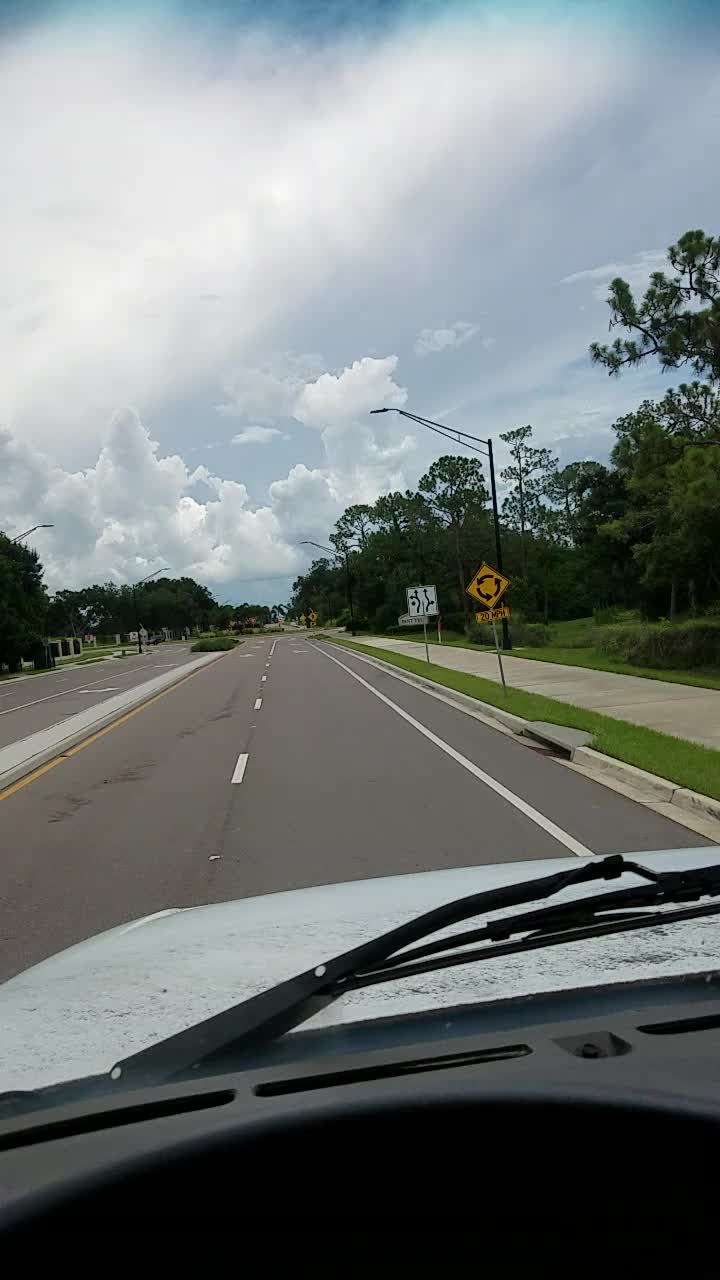This full-colour photograph captures a scenic view from inside a vehicle, focusing outward from the dashboard, which is shrouded in shadow at the bottom of the frame. The white bonnet of the car and the windscreen wipers are prominently visible. The grey road ahead features a broken white line in the center and an unbroken white line towards the right, indicating a divide between lanes.

On the left side of the road, a thin pavement separates the driving surface from a yellow-bordered area, potentially a cycle lane. To the right, there is an additional pavement edge adorned with a strip of grass. A yellow road sign stands along this edge, though its text is illegible. A smaller, white road sign is positioned behind the yellow one.

The scene is lined with trees on both sides, with those on the right appearing taller. Streetlights are visible, towering over the trees. The sky above is a mix of patches of blue and scattered clouds, adding to the tranquil atmosphere. Notably, there are no other vehicles visible on the road, contributing to the serene setting.